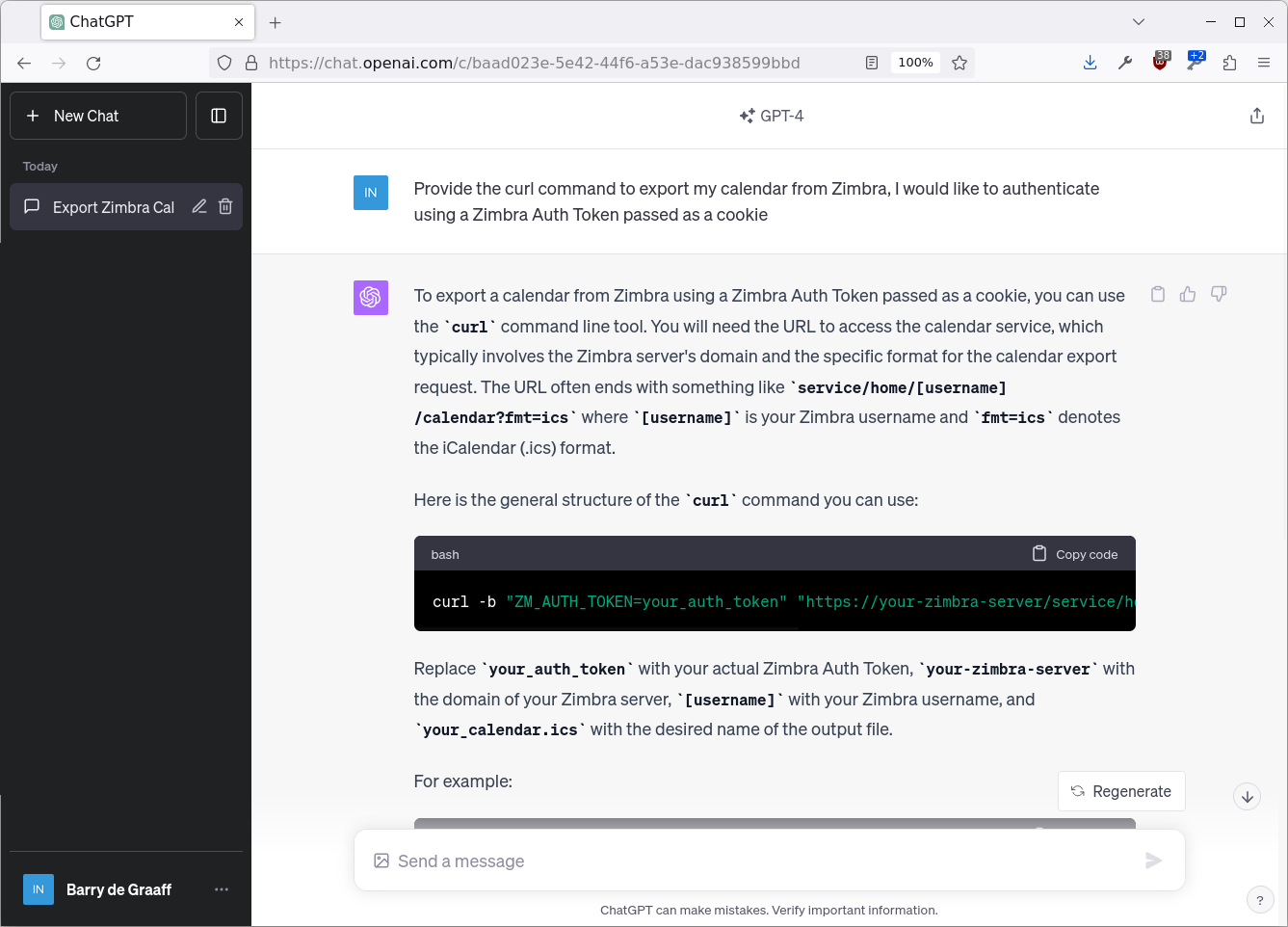The image depicts a chat interface with OpenAI's ChatGPT displayed in the top-left corner of a browser tab. The URL in the address bar reads "https://chat.openai.com". On the left-hand side of the interface, there is a vertical black sidebar containing several labeled options: "+ New Chat", "Today", "Export", and "Zimbra", followed by the icons for editing and trashing items. 

At the very bottom of the sidebar, the text "Very Deep Graaf" can be seen. The main content area of the screen shows a conversation with ChatGPT-4, where the user has asked, "Provide the curl command to export my calendar for Zimbra. I would like to authenticate using Zimbra auth token password as a cookie."

Furthermore, the response continues with: "To export a calendar from Zimbra using Zimbra auth token pass as a cookie, you can use the curl command line tool. You will need the URL to access the calendar services, which typically involves the Zimbra server domain and a specific format for the calendar export request. The URL often ends with something like '/services/home/[username]'."